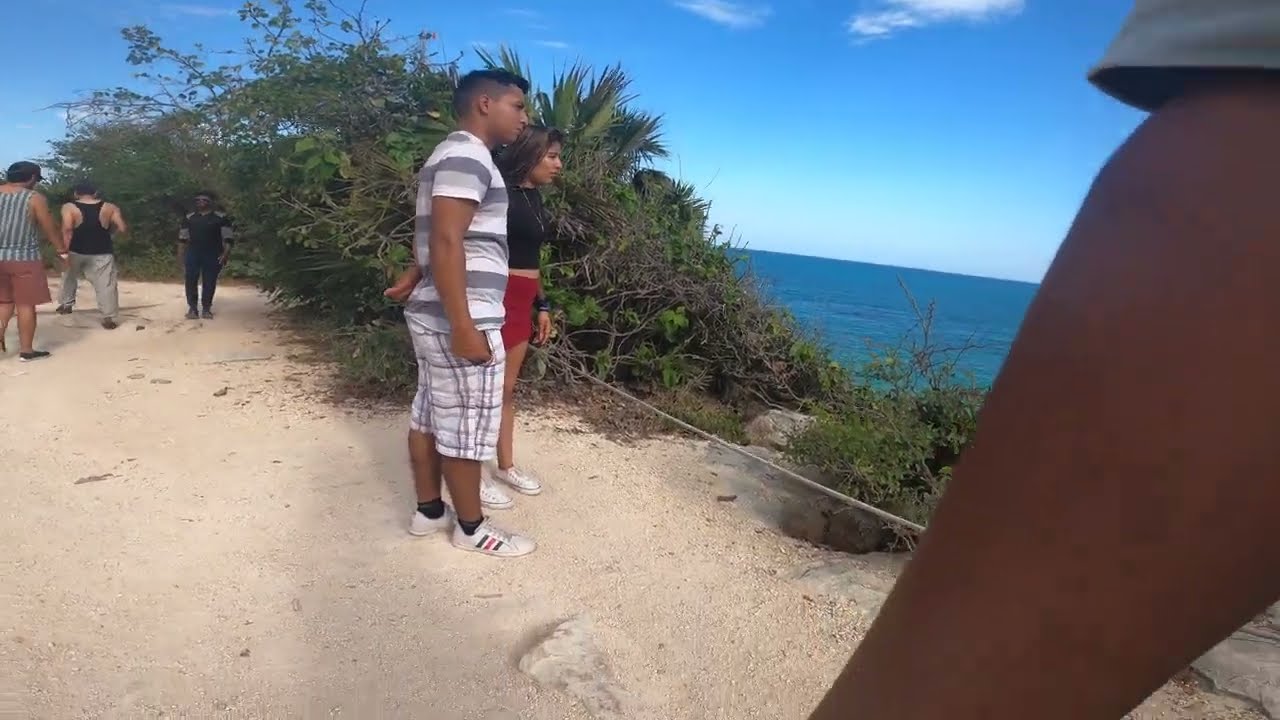In this horizontally aligned rectangular picture, a man and a woman stand near the center, gazing out over a body of water that appears to be part of the ocean. The man, who has very short black hair with shaved sides, is dressed in a gray and white striped polo shirt, gray and white plaid shorts, and white Adidas shoes. The woman beside him, visible from the side, wears a black crop top, a red miniskirt or shorts, and white tennis shoes. She has shoulder-length dark brown hair and is accessorized with a black necklace. Both individuals have slightly dark skin, suggesting they might be Latino or Asian.

They are positioned behind a low rope barrier that defines the edge of the overlook. The water ahead is dark blue and gray, while the sky is a clear blue with wispy, feathery clouds. To their left, tall green bushes with spiky leaves create a natural boundary. In the upper left corner of the image, three more people are visible, including an African-American man in a black tank top, walking on a light brown, sandy, or gravel surface. One individual’s arm, partially cut off, appears on the right side of the image. The overall setting is outdoors, likely midday, offering a serene view of nature and the ocean below.